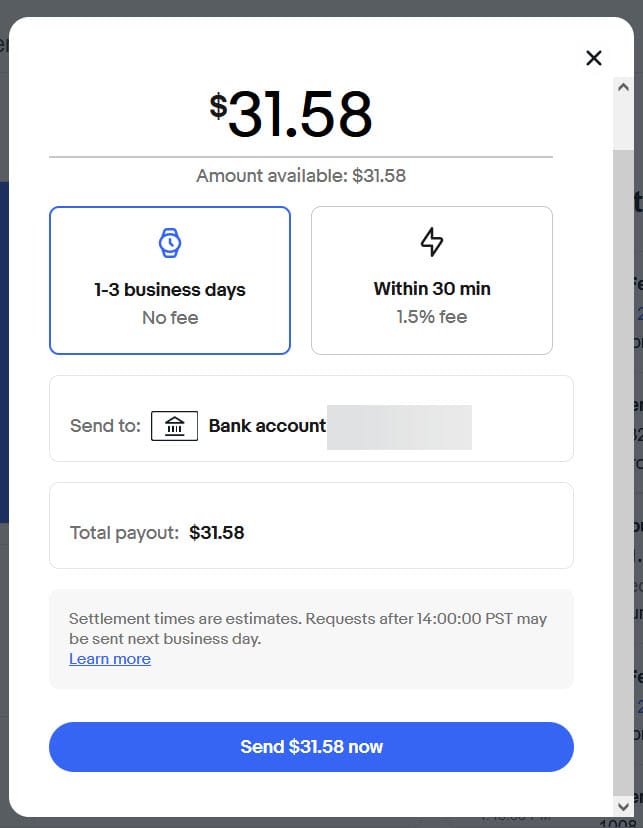This image is a detailed screenshot of a PayPal account interface. At the top of the screenshot, the balance of $31.58 is prominently displayed, noted as the "amount available." Below this, there are options for withdrawing the funds: either within one to three business days with no fee or within 30 minutes for a 1.5% fee. The withdrawal destination can be chosen, such as a linked bank account, with the total payout clearly shown as $31.58. A disclaimer states that settlement times are estimates and that requests made after 14:00 Pacific Time may be processed the next day, with a link provided for more information. At the bottom of the screenshot, there is a clickable button labeled "Send $31.58 Now" to proceed with the withdrawal. Although PayPal is not explicitly mentioned, the graphical user interface is unmistakably similar to that of PayPal, indicating that the recipient is about to withdraw $31.58 from their account.